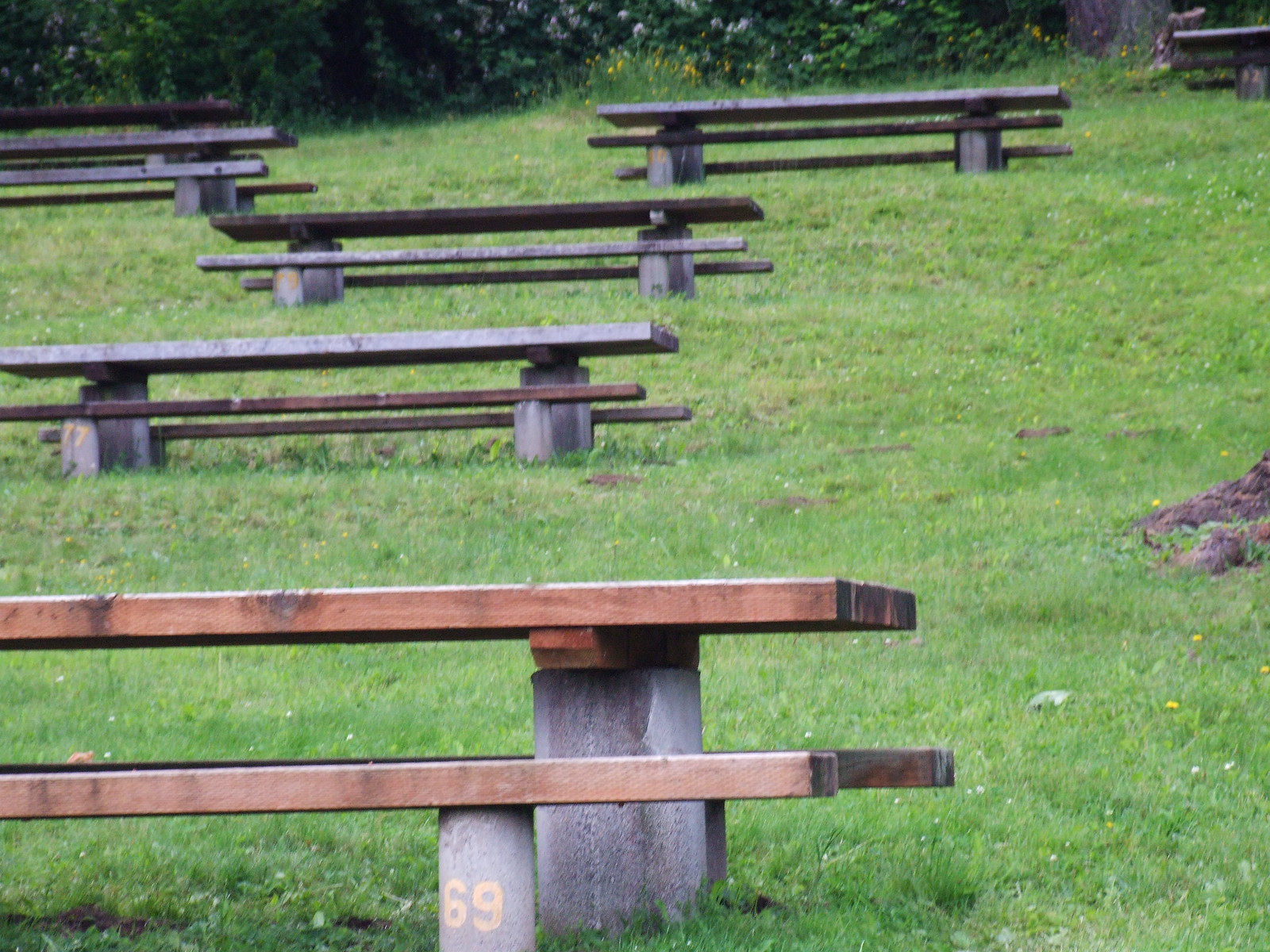The image depicts an outdoor picnic area situated on a grassy hill with a variety of trees and shrubbery in the background. There are six picnic tables scattered randomly across the grassy hillside, each supported by concrete foundations. The tables consist of thick wooden plank tabletops with matching wooden seats. Notably, one of the tables in the forefront is marked with the number 69. Additionally, a tree root is visible protruding from the ground on the right side of the image, adding a natural, rustic touch to the scene.